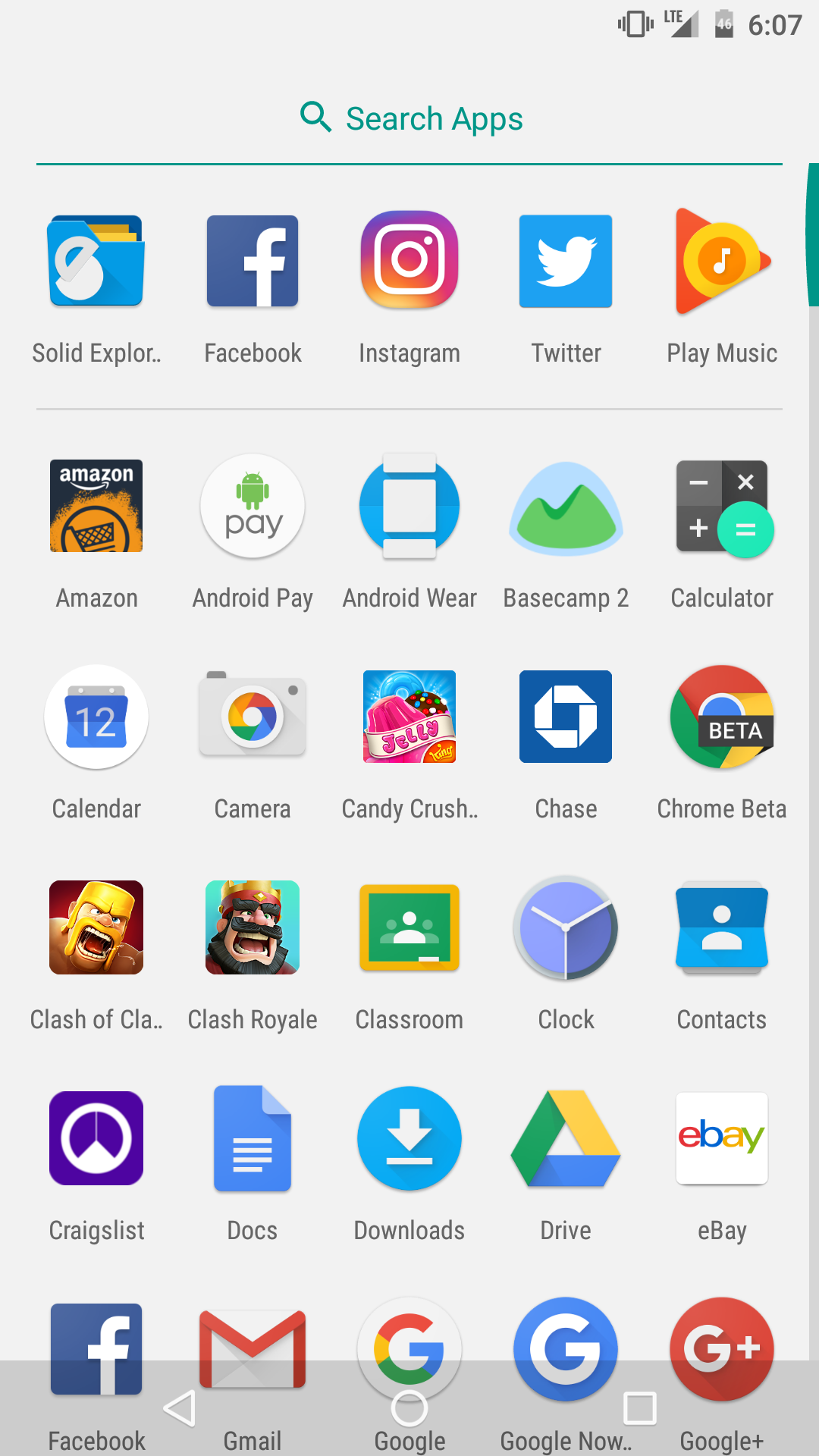This image depicts a smartphone screen displaying a grid layout of app icons within an app searching interface. At the top of the screen, there is a search bar where users can look for specific apps. Below the search bar, five app icons are arranged horizontally in a row, spanning multiple rows. The top-most row features the following apps: "Solid Explorer" (with part of the name truncated), Facebook, Instagram, Twitter, and Play Music. Each app icon is located directly above its corresponding app name.

Above this grid of apps, a thin green line is visible, accompanied by a vertical slider on the right-hand side, which allows users to scroll through the app list. Below the green line, the screen shows additional rows of app icons, organized in the same five-app-per-row layout.

At the very bottom of the screen, there is a semi-transparent, grey bar housing three navigation icons: a sideways triangle (Back), a circle (Home), and a square (Recent Apps).